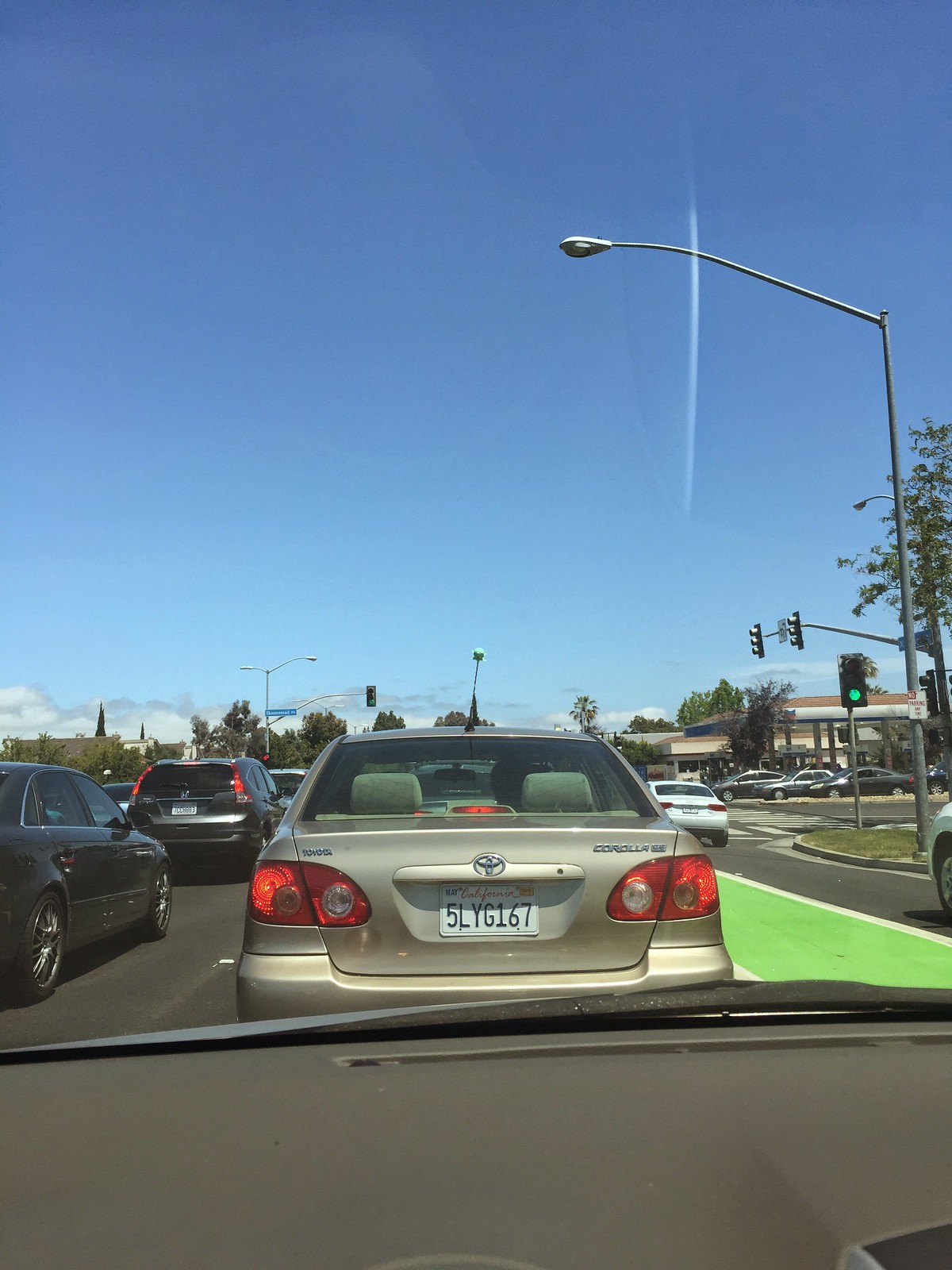The image depicts a busy road scene captured from the dashboard camera of a car. The vantage point is from just above the steering wheel, with a dark gray dashboard and a hint of the car's light silver or gray hood visible at the bottom edge. Directly ahead, there is a gold-colored Toyota Corolla with a California license plate reading 5LYG167. The Corolla's brake lights are illuminated, and it is marked with the Toyota logo and "Corolla SE" in silver letters on the rear. Surrounding the Corolla are multiple cars, with two distinctly visible to its left and others partially seen behind it, all situated at an intersection. To the right of the road is a bike lane marked with white lines, and beyond it, another road runs parallel, separated by a divider. Overhead, a street light extends over the main road. Further in the background, a gas station is discernible on the right side, while a church, partially obscured by trees, can be seen to the left. The sky above is bright blue with some hazy clouds, indicating daytime. Traffic lights at the intersection suggest that the light may have just turned green, with the vehicles preparing to move forward.